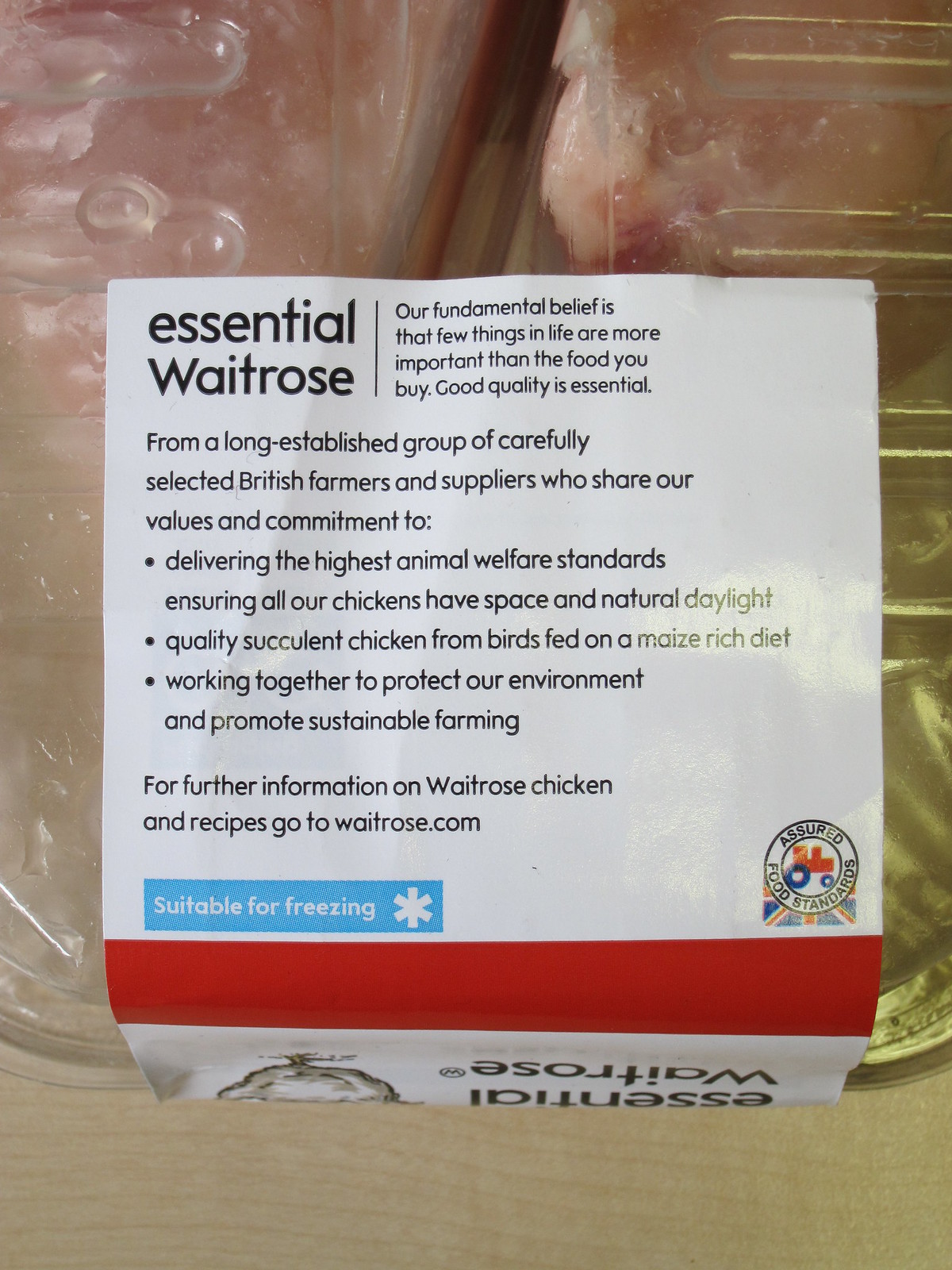This photograph captures a detailed close-up of a white label on a clear plastic packaging containing pinkish pieces of meat, likely chicken. The large white label dominates the image, extending down the side and top of the packaging. The top left of the label prominently displays the text "Essential Waitrose" in bold black letters, with only the 'W' capitalized. Adjacent to this on the right is a statement: "Our fundamental belief is that few things in life are more important than the food you buy. Good quality is essential."

Below this, a column of text reads: "From a long-established group of carefully selected British farmers and suppliers who share our values and commitment to delivering the highest animal welfare standards, ensuring all our chickens have space and natural daylight. Quality, succulent chicken from birds fed on a maize-rich diet. Working together to protect our environment and promote sustainable farming."

Continuing downward, the label advises: "For further information on Waitrose chicken and recipes, go to waitrose.com." A light blue rectangle at the bottom right features the words "Suitable for freezing" in white, accompanied by a snowflake symbol.

Near the bottom right corner of the label, there is a small logo incorporating the British flag in black, blue, and red. Beneath this, a large red banner stretches horizontally across the label. Below the banner, some additional text is visible but partially obscured due to the bag's positioning.